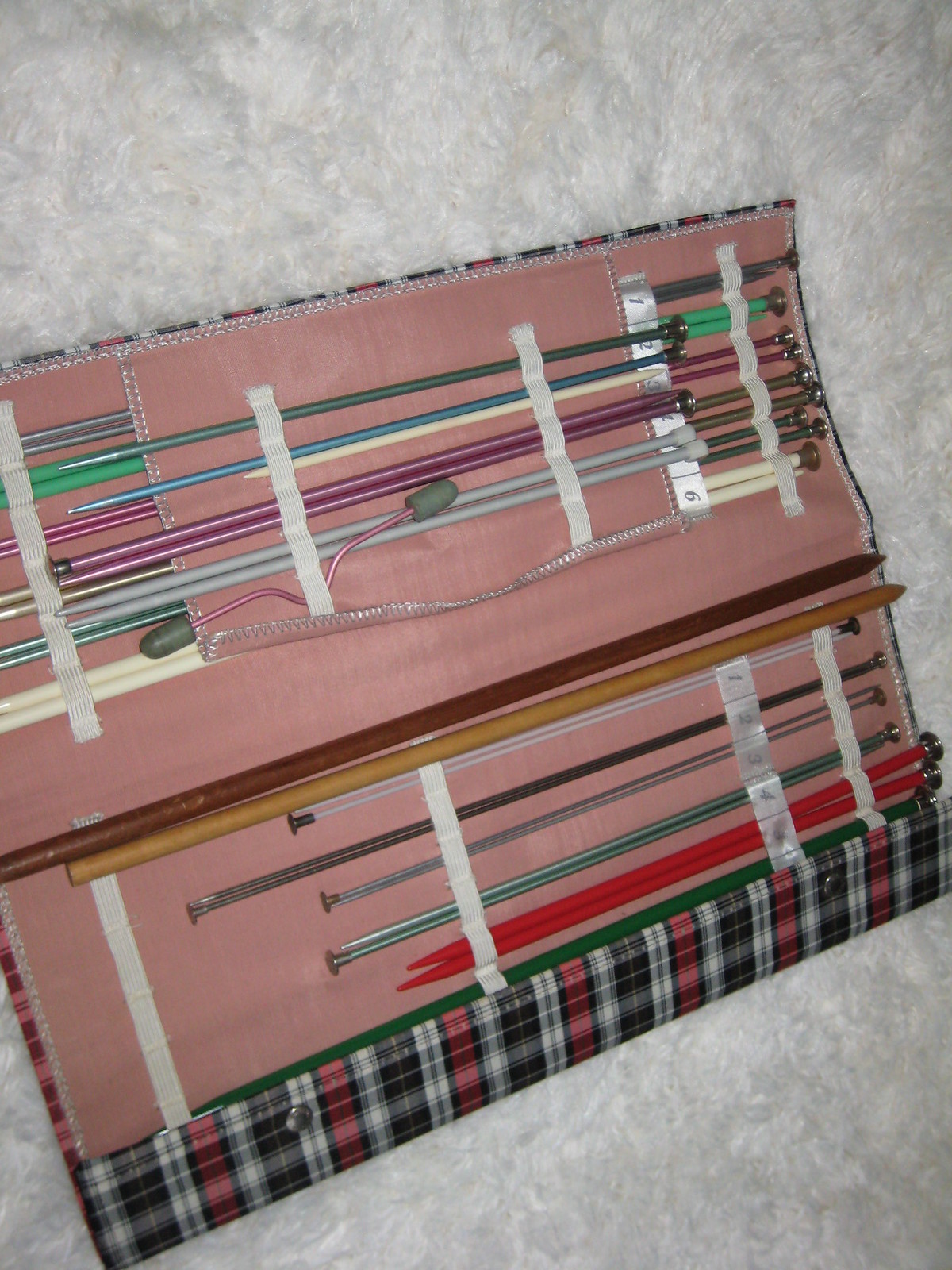This image captures a handmade knitting needle case displayed on what appears to be a fluffy white surface, possibly a blanket or a carpet. The case, which has a red, white, green, and gray plaid exterior, is open to reveal both its top and bottom sections. Inside, the case is lined with a dusty pinky rose material and features white elasticated straps to hold the tools securely in place. The assorted knitting needles come in various sizes and styles, including sets of red, silver, and wooden needles, as well as a specialized needle for knitting rounds or sleeves. This detailed and well-organized knitting kit, reminiscent of the ones used by grandmas for crocheting, showcases essential tools and needles neatly arranged, emphasizing its practical and handcrafted charm.